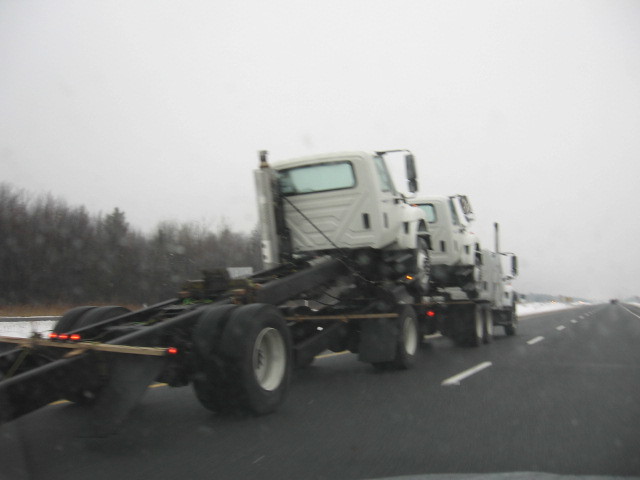In this image, we see a winter scene on a highway that appears to be slightly uphill. The sky is a light, overcast gray without visible clouds or sunlight, enhancing the desolate atmosphere. Snow is scattered on the ground beside the black asphalt road, which features white dashed lines in the middle and yellow lines along the sides. On the left side of the road, dense, dark trees devoid of leaves add to the wintry feel.

A large white truck is prominently in view, traveling in the left lane of the seemingly long and empty highway. This truck, resembling a semi but without a trailer attached, has a flatbed hauling two more identical white truck cabs. Each vehicle is equipped with large, wide tow mirrors, exhaust stacks, and big tires. The truck ahead in the distance is the only other vehicle visible on this quiet, gray day.